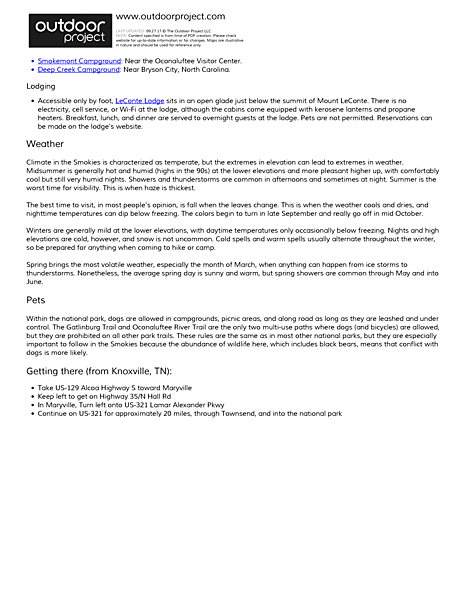The image depicts a web page accessed on a smartphone, featuring the "Outdoor Project" website. Positioned at the top of the page, left-justified, is a stylized logo: "Outdoor" in white lowercase letters above "project" in light green lowercase letters, right-justified within a black box. To the right of this logo, the URL www.outdoorproject.com is displayed, accompanied by a brief tagline.

Below the logo, in blue text, the webpage provides information about various campgrounds near notable landmarks. Though some of the names are difficult to read due to their length or complexity, one clearly identifiable location is Deep Creek, near Bryson City, North Carolina. Users have the option to click on these campground links for more details.

Further down, a section titled "Lodging" appears, rendered in gray letters on a white background. This section describes La Conte Lodge, accessible only by foot and set in an open glade just below the summit of Mount La Conte. The lodge offers a rustic experience, with no electricity, cell service, or Wi-Fi. Instead, cabins are furnished with kerosene lanterns and propane heaters. Meals are provided for overnight guests, but pets are not allowed. Reservations must be made through the lodge's website.

Additional details about the lodge cover weather conditions, further elaboration on the pet policy, and directions on how to reach the lodge from Knoxville, Tennessee—suggesting that the user accessing this web page might be located in or planning a trip from Knoxville. This comprehensive page serves as a useful resource for those looking to immerse themselves in nature at La Conte Lodge.